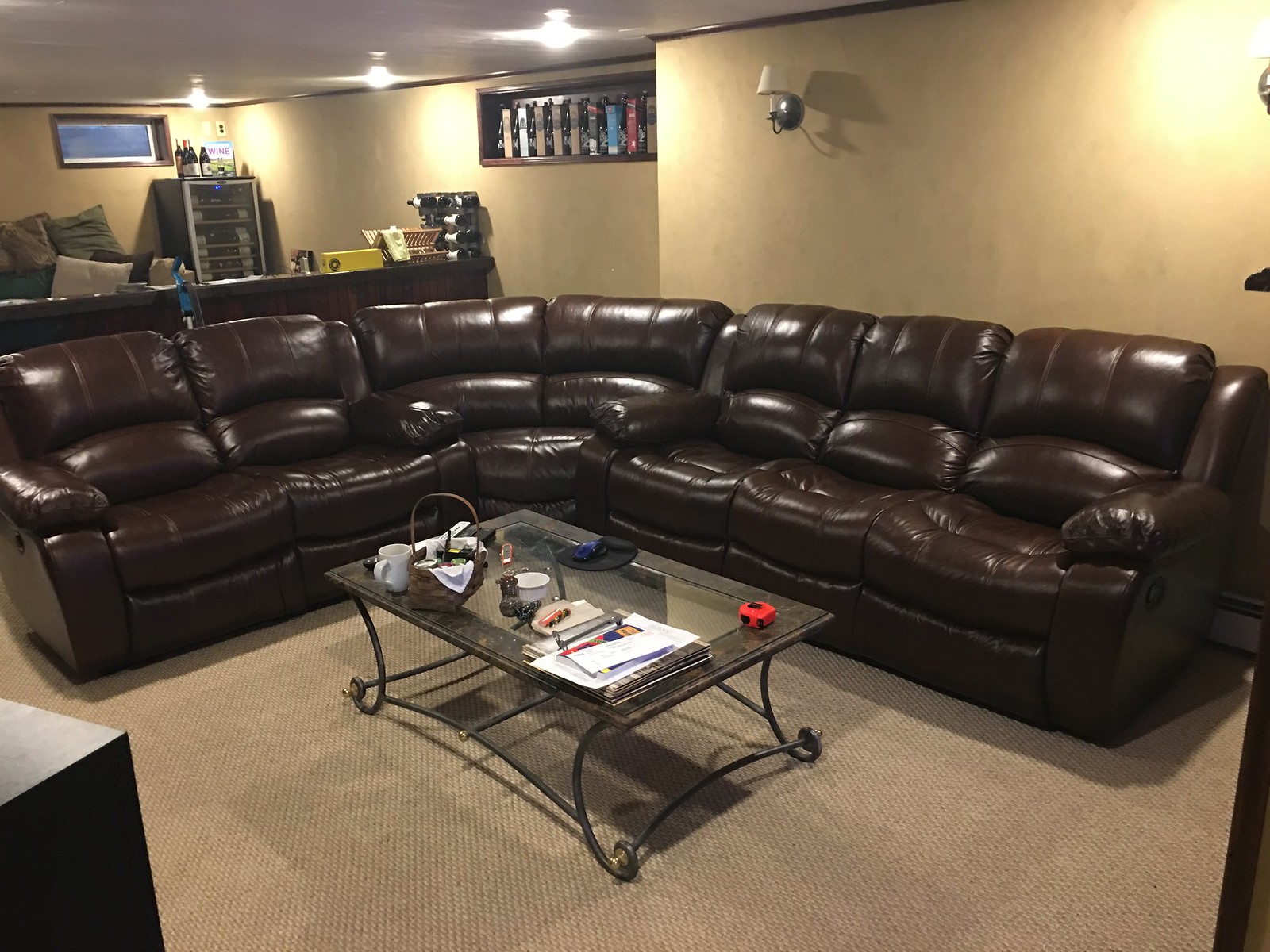The image depicts what appears to be a cozy basement living area. Dominating the scene is a large, dark brown leather sectional sofa arranged in a U-shape with a noticeable curve, giving it an L-shaped appearance. The sofa is shiny and spacious, suggesting it may have recliner features. In front of the sofa sits a glass and metal coffee table, laden with various items: a basket, a white mug, some papers, a red tape measure, and a white bowl.

The room's flooring is a beige carpet, complementing the beige and slightly yellow-toned walls. Several light sconces are mounted on the walls above the sofa, providing localized lighting, while additional ceiling lights illuminate the area. In the background, to the left, there's a small cubby or bar area featuring a wine cooler with some wine bottles and a stack of couch pillows. A small rectangular window is set high on the back wall, offering a view of something blue outside. A brown shelf is also visible on the wall, possibly holding awards or other items, adding to the room's detailed coziness and functionality.